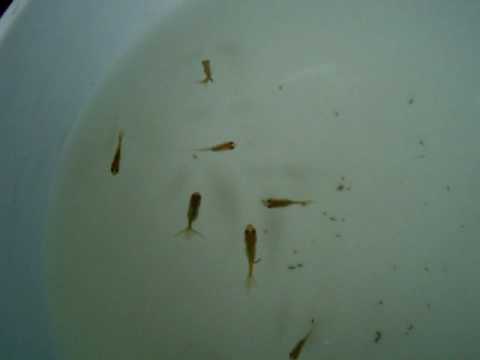This is an overhead photo of a white bowl filled with slightly murky water, showcasing seven tiny, brownish, fish-like creatures swimming in various directions. The bowl's curved edge is visible in the upper left-hand corner. The water has a subtle greenish tint in the center and contains several small, dark specks—possibly dirt, waste, or smaller, indistinguishable fish. Each fish has an oblong body that thins into feathery tails, suggesting they are too small for consumption and likely intended as pets or for observational purposes.